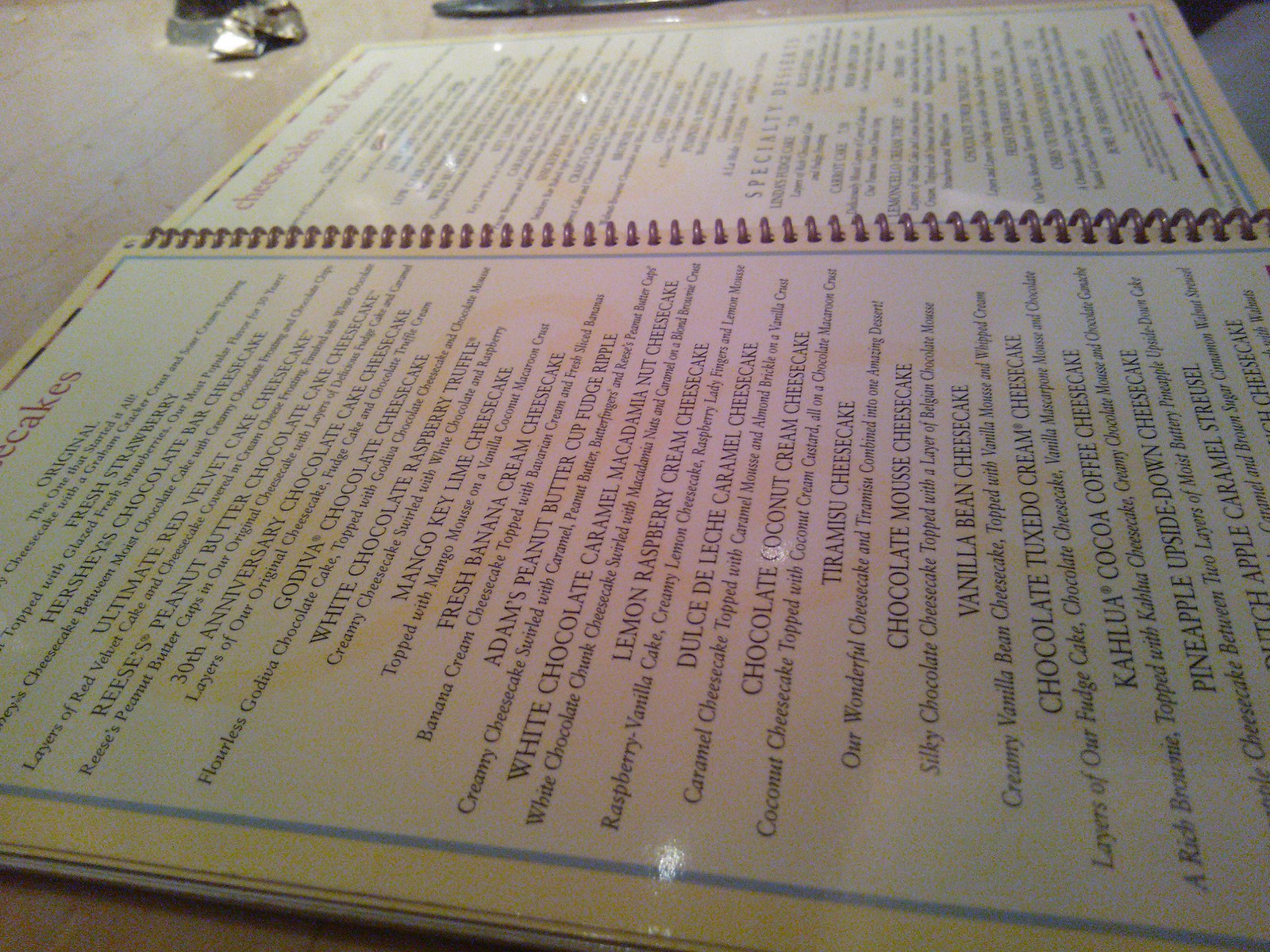Captured at an angle, this image showcases a spiral-bound menu opened to its dessert section. The menu binding, a reddish-brown spiral, runs horizontally across the picture. To read the contents, one would need to turn the picture sideways. The menu prominently features an extensive selection of cheesecakes, suggesting either a specialty cheesecake store or a dedicated dessert section.

Featured cheesecakes include:
- Original
- Fresh Strawberry
- Hershey's Chocolate Bar Cheesecake
- Ultimate Red Velvet Cake Cheesecake
- Reese's Peanut Butter Chocolate Cheesecake
- 30th Anniversary Cheesecake
- Godiva Chocolate Cheesecake
- White Chocolate Raspberry Truffle
- Mango Key Lime Cheesecake
- Fresh Banana Cream Cheesecake
- Adam's Peanut Butter Cup Fudge Ripple
- White Chocolate Caramel Macadamia Nut Cheesecake
- Lemon Raspberry Cream Cheesecake
- Dulce de Leche Caramel Cheesecake
- Chocolate Coconut Cheesecake
- Tiramisu Cheesecake
- Chocolate Mousse Cheesecake
- Vanilla Bean Cheesecake
- Chocolate Tuxedo Cream Cheesecake
- Kahula Cocoa Coffee Cheesecake
- Pineapple Upside-down Cheesecake
- Apple Caramel Streusel

The other page in the background is visible but the text is too blurred to read.